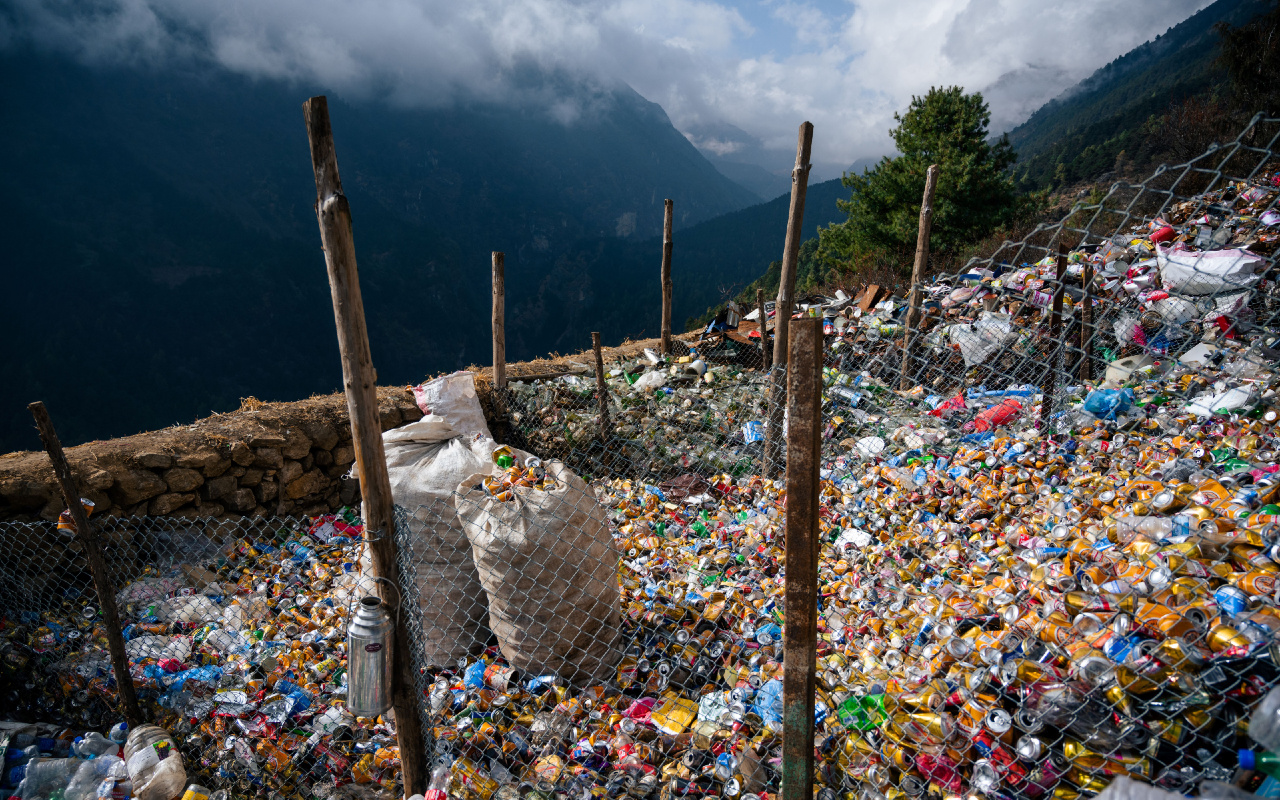The image depicts a striking contrast between a garbage dump and a beautiful natural landscape. In the foreground, a large amount of trash, predominantly aluminum cans, is piled up inside a fenced area. The fence comprises chain link or chicken wire supported by tall wooden posts, with a noticeable thermos hanging from the tallest post on the left side. Scattered among the cans are two large sacks of refuse, positioned towards the left and center of the image. The fenced area sits on an incline, with different sections filled with various types of garbage, including trash bags and miscellaneous refuse. Descending into the background, the scene transitions into a serene natural setting featuring a tree on the right, rolling hills, and a majestic mountain range under a vast sky filled with white clouds. The juxtaposition of the polluted foreground against the pristine, scenic background evokes a sense of environmental disarray and raises questions about waste disposal practices, possibly in a location reminiscent of places like Thailand or India.